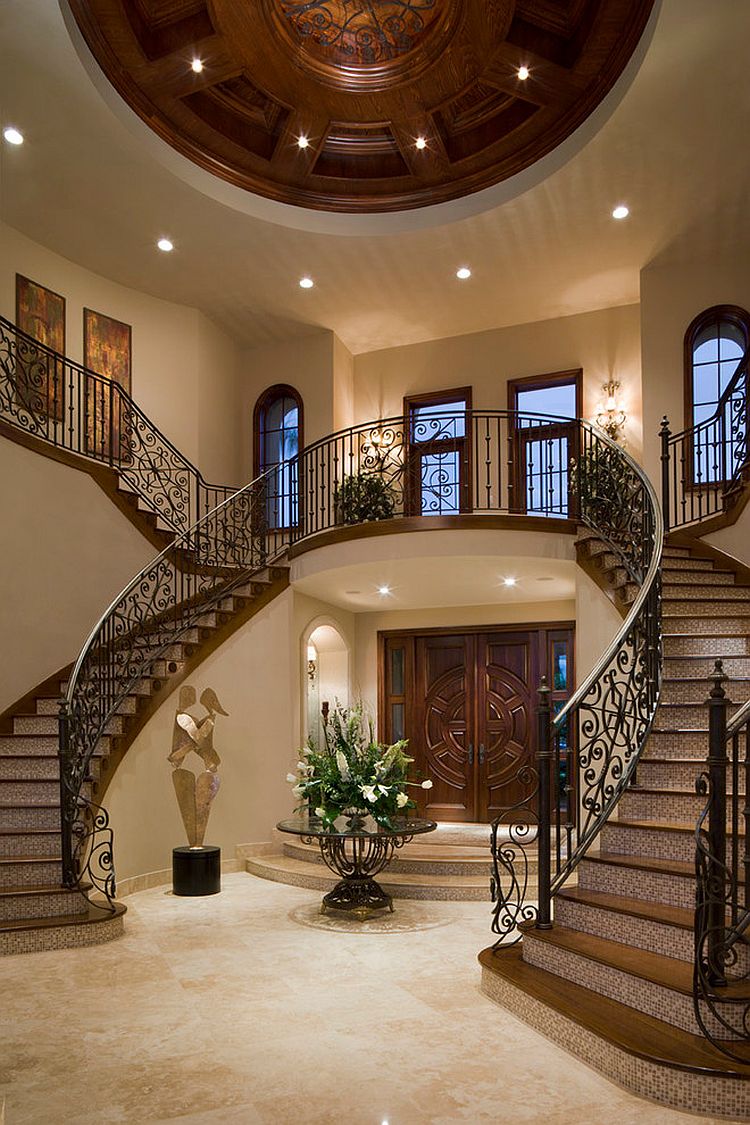This is the inside view of a grand mansion's main entrance, exuding opulence and architectural splendor. At the forefront, a pair of imposing double doors stands as a gateway, welcoming guests into the vast, well-lit space. Directly ahead of the entrance is an intricately crafted table adorned with an expansive flower pot, overflowing with vibrantly colored blooms, adding a touch of nature's elegance to the lavish interior. To the left of the floral arrangement, a small, exquisitely detailed statue stands as a testament to fine artistry.

A grand staircase ascends to a raised platform directly above the main doors, serving as a focal point in this magnificent space. From this elevated point, two additional broad staircases branch out symmetrically, each extending upwards and providing access to higher levels of the mansion. The ceiling above the entrance showcases a majestic dome, intricately designed and accentuated by a series of recessed lights arranged in a circular pattern, casting a soft, ambient glow throughout the hall. The overall composition of the entrance hall combines classical elegance with contemporary design, making it an awe-inspiring introduction to the grandeur that lies within the mansion.